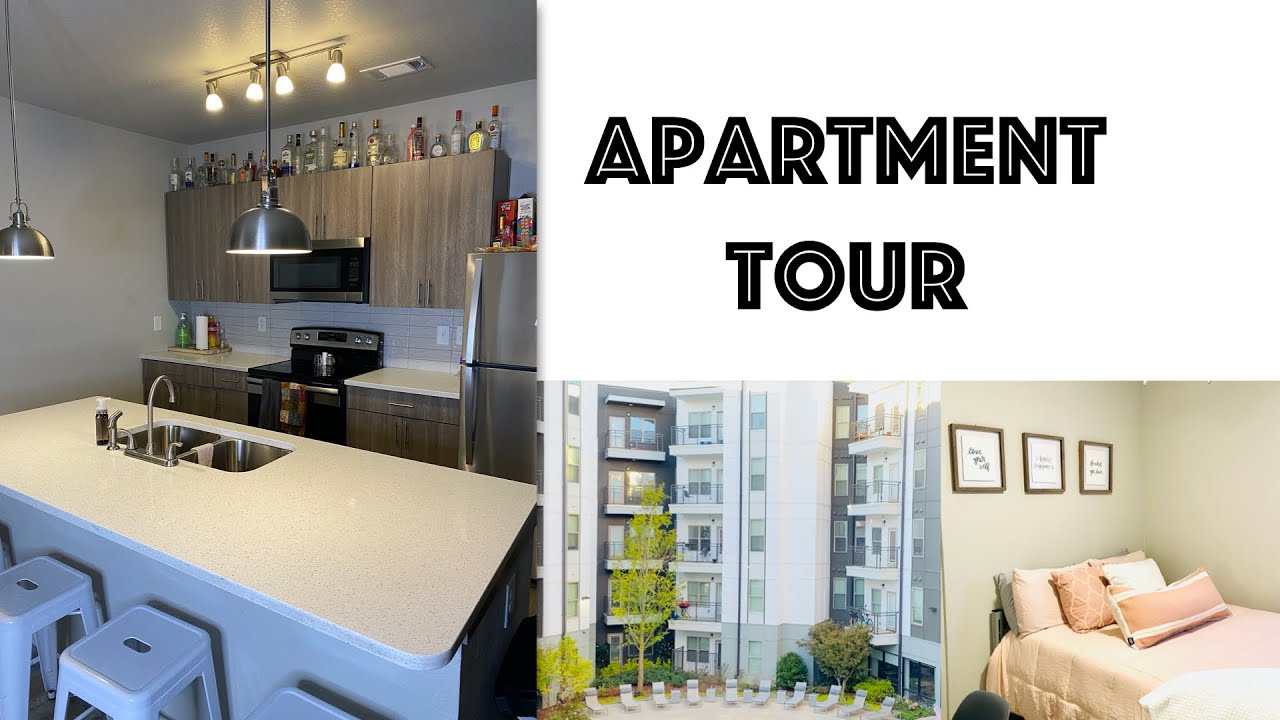The image is a collage of photos showcasing an apartment tour. 

On the left, we see the interior of a modern kitchen. The kitchen features white walls and ceiling, complemented by track lighting and two sleek, silver metallic pendant lights hanging above the center console. The console itself boasts white speckled synthetic countertops, two metallic sinks, and plastic bar stools. In the background, there are minimalist cabinets, a prominent stainless steel fridge, and a black stove centrally located. The area around the range and stove is adorned with several bottles of alcohol and is set against a light gray tiled backsplash. Additional items are placed on top of the fridge, completing the kitchen's lived-in look.

On the top right of the collage, bold capital letters with thin white lines inside them spell out "APARTMENT TOUR." 

Below this text, there are two more photos. The first depicts the exterior of the apartment building. The facade features a mix of dark gray, white, gray, and black colors arranged in varying shades and non-linear angles, giving it a dynamic and contemporary appearance. In front of the building, shades and lounges are arranged in a curved pattern, possibly by a pool which is not visible in the photo.

The second photo on the far right shows a cozy bedroom. Above the simple bed frame, three framed square photos are arranged neatly. The bed is adorned with a pink blanket and is piled high with five stacked pillows, creating an inviting and comfortable atmosphere.